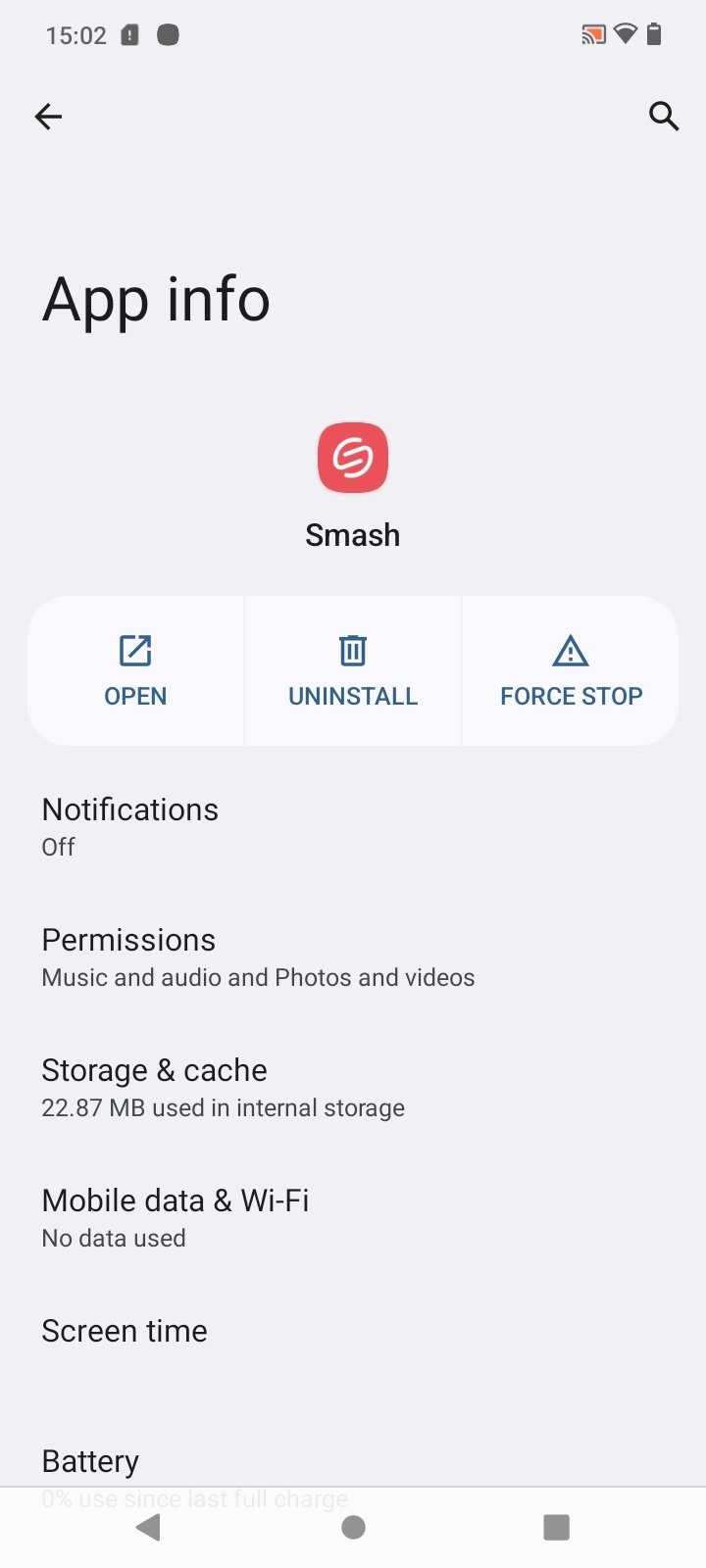This image is a detailed screenshot from a mobile phone displaying the app information screen for the "Smash" app. The background is a light gray color. 

At the very top, displayed in black text, the time reads 15:02. To the right of the time, there are icons indicating the phone's status: an SD card icon, a black circle icon, a Wi-Fi icon with full signal bars, and a full battery icon. 

Below this status bar, on the left side, there is a small black left-pointing arrow, and on the right, a small black magnifying glass icon, likely for search purposes.

Next, in larger text, it says "App info" followed by the app's logo: a red square with a white speech bubble containing a stylized 'S'. Directly below this logo, the app name, "Smash," is written in black font.

Further down, there is a white oval segmented into three parts. On the left section is an icon of a square with an arrow, labeled "Open." In the middle section, there is a trash can icon labeled "Uninstall." The right section displays a triangle with an exclamation point at its center, labeled "Force stop."

Beneath this, in black font, it states "Notifications off." 

Following this, a list of permissions granted to the app is given: "Music and audio" and "Photos and videos."

The storage usage is displayed next: "Storage & cache - 22.87 MB used in internal storage."

At the bottom of the image, it reads: "Mobile data & Wi-Fi."